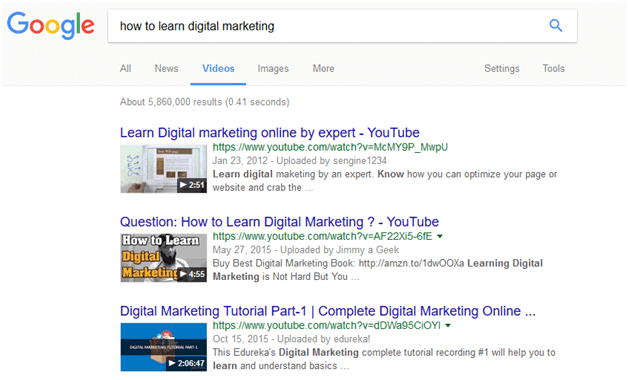The image displays a Google search results page for the query "how to learn digital marketing." In the upper left corner, the colorful "Google" brand logo is prominently visible with the following sequence of colors: a blue "G," a red "O," a yellow "O," a lowercase blue "g," a green "l," and a red "e." To the right of the logo is the search bar with the text "how to learn digital marketing" entered, and the blue search magnifying glass icon at the far right of the bar. This entire section is set within a light gray header panel.

Below the header, the search results are organized into five tabs: "All," "News," "Videos," "Images," and "More." The "Videos" tab is currently selected and highlighted in blue with a blue underline, indicating that video results are being displayed. The unselected tabs "All" and "News" are to the left of "Videos," while "Images" and "More" are to the right, all in light gray. The "Settings" and "Tools" options, also in gray, are positioned at the far right of the tab row.

In the main body of the search results, gray text informs the user that there are approximately 5,860,000 results found in 0.41 seconds. The first three video results are displayed prominently. Each video result includes a blue title, a thumbnail image, a green URL, the upload date, and a brief description:

1. **Learn Digital Marketing Online by Expert - YouTube**
   - Thumbnail: A laptop screen displaying a marketing page.
   - URL: YouTube link
   - Upload Date: January 23, 2012
   - Uploaded by: Sengen1234

2. **How to Learn Digital Marketing - YouTube**
   - Thumbnail: Generic YouTube bubble text with "how to learn" in white and "digital marketing" in orange.
   - URL: YouTube link
   - Upload Date: May 27, 2015
   - Uploaded by: JimmyAGeek

3. **Digital Marketing Tutorial - Part One | Complete Digital Marketing...**
   - Thumbnail: A blue background with a box icon and an illegible black text box above it.
   - Duration: 2 hours, 6 minutes, and 47 seconds
   - Upload Date: October 15, 2015
   - Uploaded by: edureka!

This descriptive caption provides a detailed overview of the Google search results page, including the layout and specifics of the video results displayed.